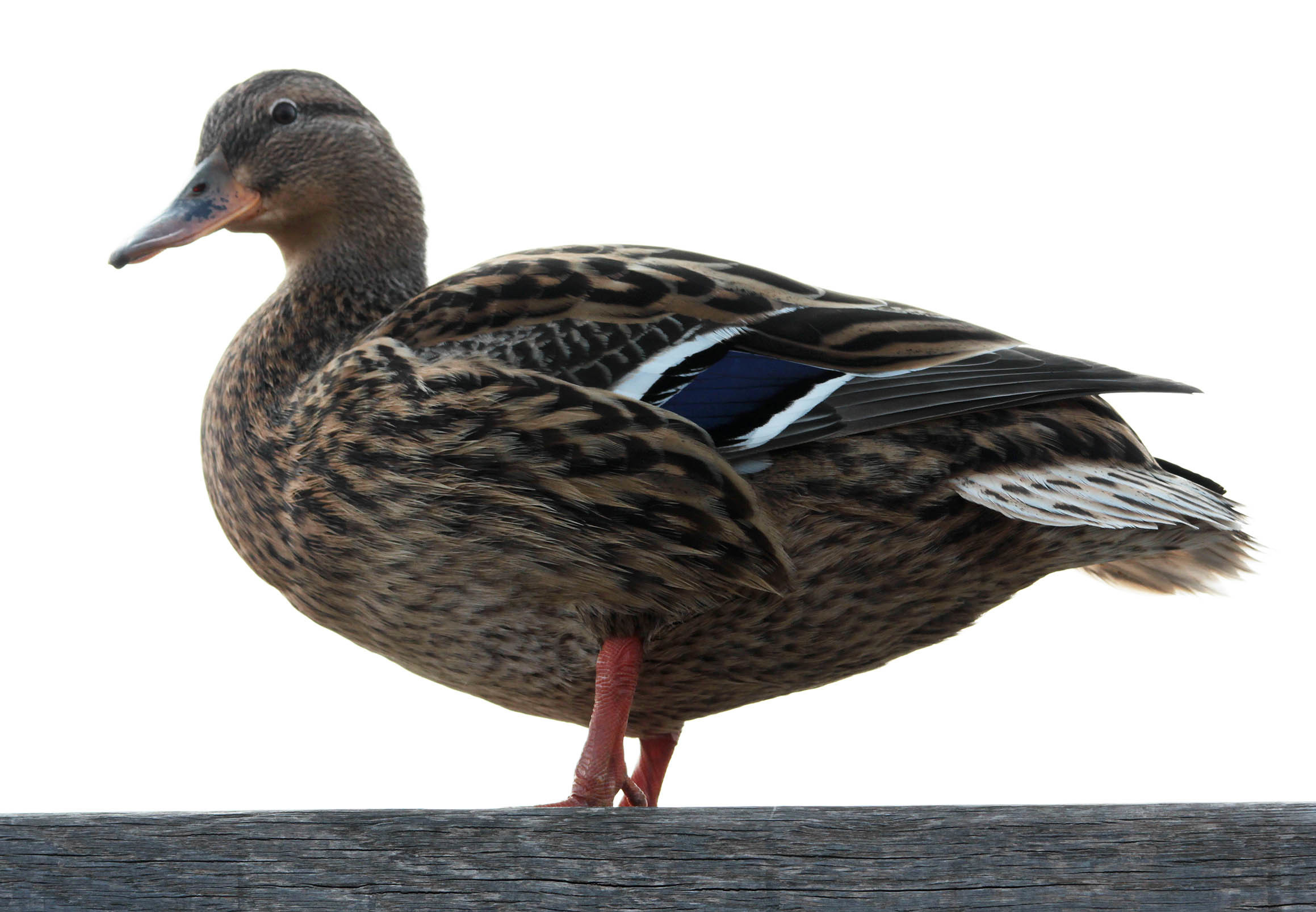The image features a single, well-fed duck standing on a horizontal piece of wood. The scene is zoomed in, providing a detailed side view of the duck, which is centered against a completely white background. The duck's body faces left, around the nine o'clock position, while its head is slightly turned towards the camera, at about the 8:30 position. It has an orange beak and its feathers are predominantly white to light brown, with black accents throughout. Distinctive under feathers in dark blue, black, and white can be seen beneath the primary feathers. The tail sports a mix of white and black feathers. The duck has large feet and a textured pattern of coloration, displaying hues of white, brown, black, orange, yellow, and gray. The piece of wood it stands on is located at the bottom of the frame, grounding the composition in an outdoor setting, possibly near a duck pond.